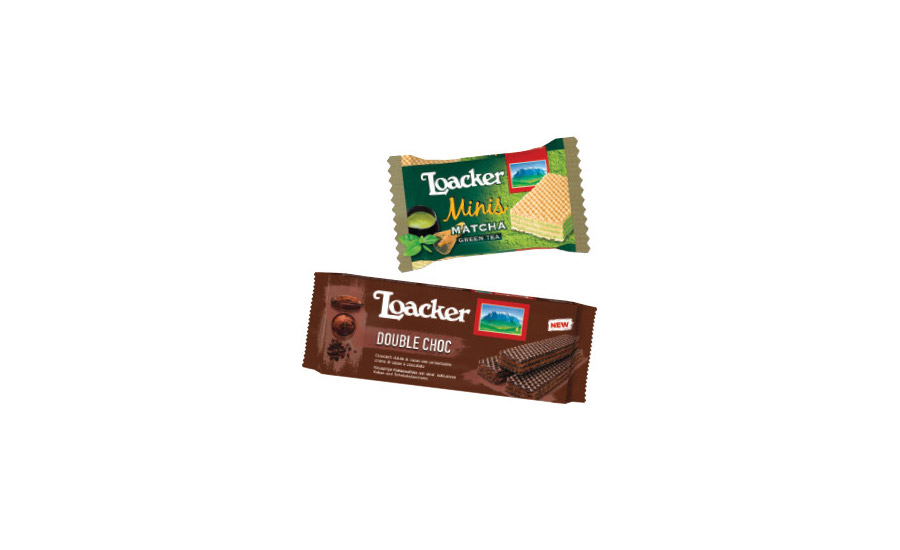This image showcases two intricately detailed packages of Loacker wafers. The top package, smaller in width, features a green wrapper denoting the "minis matcha green tea" flavor, with an illustration of a light beige wafer with green tea filling. To the left of the wafer image, there are pictures of tea leaves, accentuating the matcha theme. The perforated edges of this pack indicate easy opening.

The bottom package is larger and marked with a rich, dark brown color signaling the "Double Choc" flavor. It prominently displays the Loacker logo in white, a red square with grass and mountain imagery, and a banner proclaiming "new" adjacent to drawings of cocoa beans. The visual includes brown wafers with chocolate filling, emphasizing the double chocolate indulgence. The overall packaging design effectively highlights both flavors through distinctive color schemes and detailed illustrations.